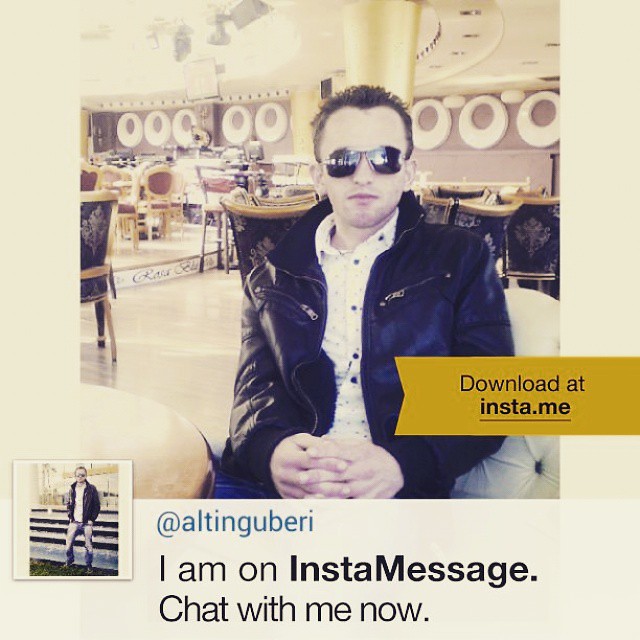This vibrant-colored image printed on cardstock features a young gentleman seated in an opulent, spacious room adorned with numerous tables and chairs, suggesting a high-end restaurant setting. He is dressed in a white shirt and layered with a substantial black leather jacket, and he dons sunglasses despite being indoors. His arms are crossed, resting in front of him in a poised manner. A prominent yellow block on the image reads "Download at insta.me," accompanied by a smaller image of the same gentleman standing outdoors in the identical outfit sans sunglasses. The text below this smaller picture prompts interaction with the message, "I am on InstaMessage, chat with me now."